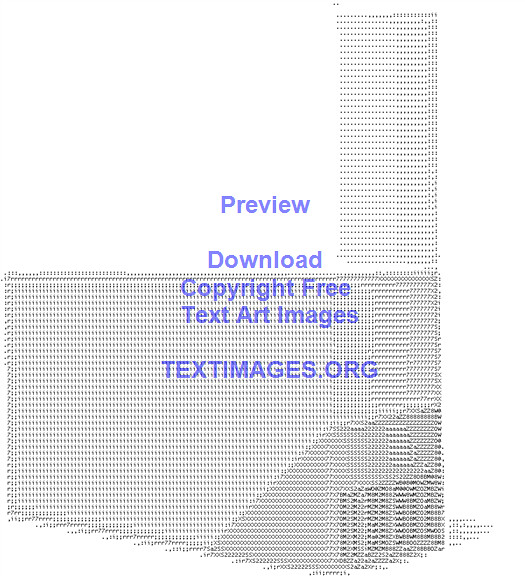This image features a detailed artwork of a digital building constructed from various letters, numbers, and characters, all set against a dominant white background. The building, which includes a prominent chimney and several doors, is intricately rendered in black text. Notable characters such as the number '2' and the letter 'M' are visible within the structure's design. Overlaying the center of the building in purple text are the words: "Preview Download Copyright Free Text Art Images," with each word's initial letter capitalized. At the bottom, the website "TEXTIMAGES.ORG" is displayed in all caps. The overall composition creates a striking black-and-white visual effect, with the purple text adding a distinct contrast.